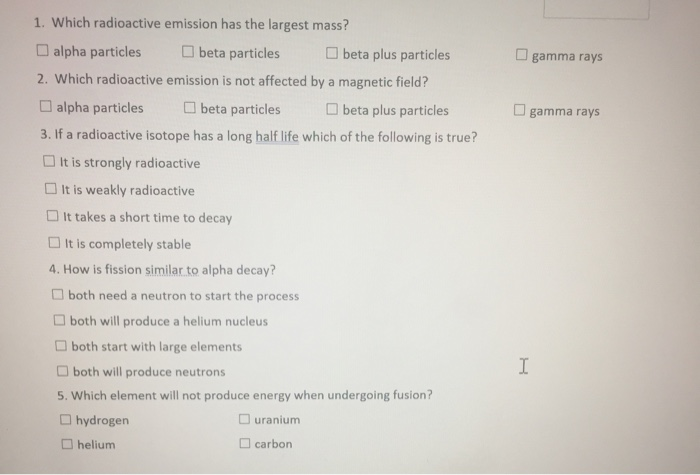This image, resembling a multiple-choice test page, features detailed questions and answer choices pertaining to radioactive emissions and nuclear reactions. 

1. **Which radioactive emission has the largest mass?**
   - Alpha particles (left)
   - Beta particles (next to the right)
   - Beta plus particles (next to beta particles)
   - Gamma rays (last option on the right)

2. **Which radioactive emission is not affected by a magnetic field?**
   - Alpha particles (front option)
   - Beta particles (next in line)
   - Beta plus particles (following beta)
   - Gamma rays (final choice)

3. **If a radioactive isotope has a long half-life, which of the following is true?**
   - It is strongly radioactive (top choice)
   - It is weakly radioactive (below strongly radioactive)
   - It takes a short time to decay (next option)
   - It is completely stable (last option)

4. **How is fission similar to alpha decay?**
   - Both need a neutron to start the process (first option)
   - Both will produce a helium nucleus (below neutron)
   - Both start with large elements (following helium nucleus)
   - Both will produce neutrons (final choice)

5. **Which element will not produce energy when undergoing fusion?**
   - Hydrogen (top option)
   - Uranium (across from hydrogen)
   - Helium (bottom option)
   - Carbon (across from helium)